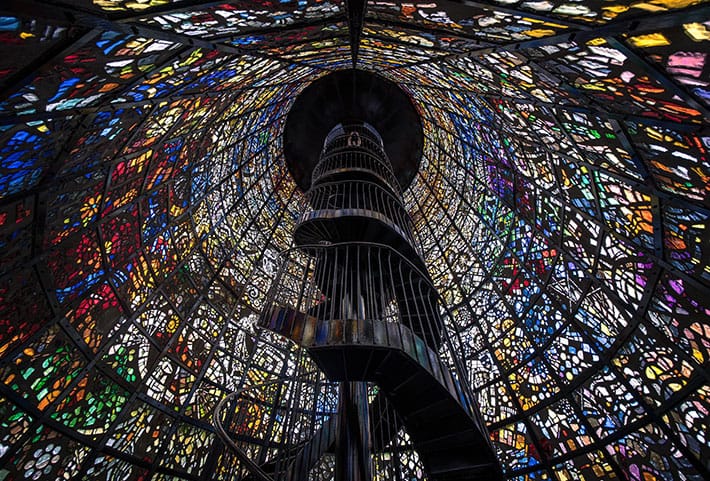The image showcases the inside of a cylindrical building with a tall, black metal spiral staircase ascending from the bottom of the frame to the top. Our perspective is from the base of the staircase, looking upwards. The structure is surrounded by an elaborate display of stained glass window panes arranged in circular patterns. These panes feature a mosaic of various colors—dominantly navy blue, red, yellow, green, white, orange, and purple—without depicting any specific characters or symbols, just abstract shapes and swirls. The staircase is adorned with railing on the sides, enhancing its intricate design. Near the center of the image, two figures are discernible on the staircase, adding a sense of scale to the imposing structure. The top of the image shows a black circular area, blending into the background, leaving the destination of the staircase unseen.